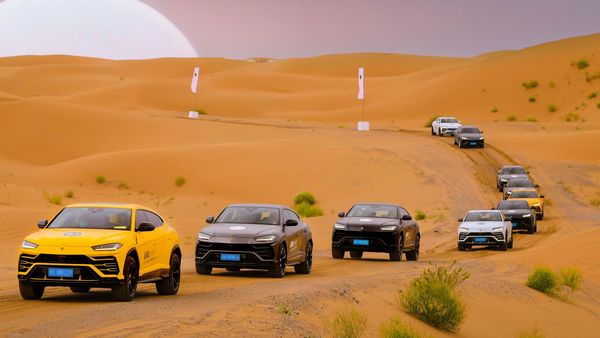The rectangular image, oriented with its long side running horizontally, captures a striking scene of a convoy of identical cars traversing a desert landscape. Anchoring the bottom left is a yellow car, followed by two grayish-black cars. Nearing the right edge of the image is a white car, with a series of four more cars continuing upward in a line. Further in the distance, closer to the middle right, two additional cars can be seen. The terrain—vast, undulating sand dunes—dominates the background, accented by sporadic green plants. Central to the scene are two flags, possibly indicating a designated path for the vehicles. Above, a grayish and white sky looms over the arid expanse, completing the dramatic and adventurous tableau.